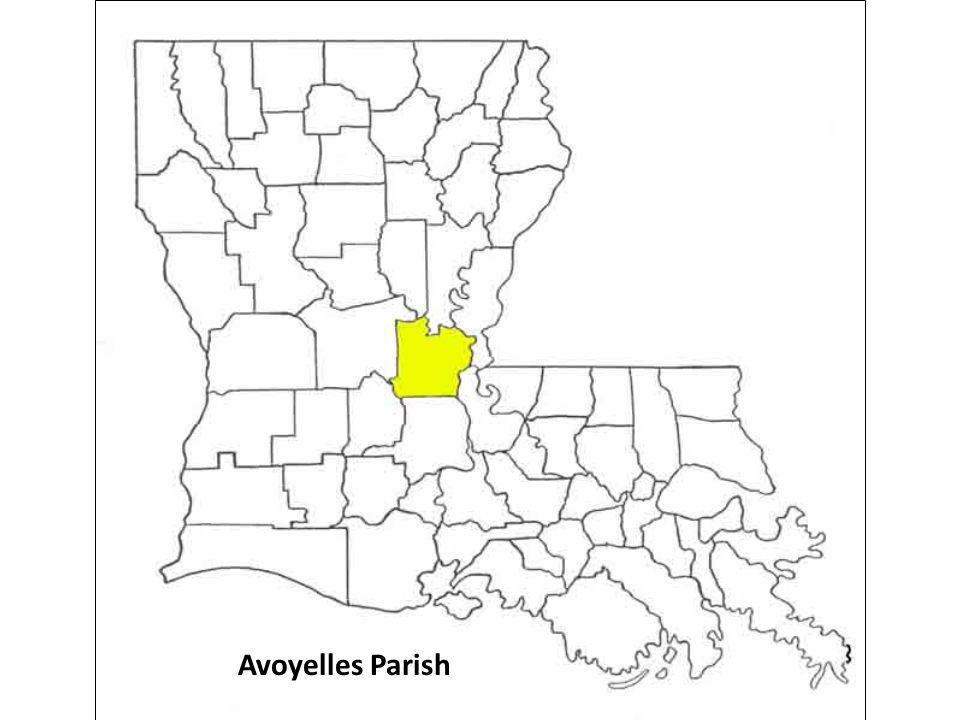This image is a detailed, black-and-white map of the state of Louisiana, displaying the precise outlines of its many parishes. Each parish boundary is intricately drawn in thin black lines against a stark white background, creating a clear and uncluttered geographical depiction. The map is enclosed within a black border, further framing the state. Notably, there is a single parish in roughly the center of Louisiana that is highlighted in yellow, distinctly standing out from the rest. This highlighted area is labeled as "Avoyelles Parish" in black font at the bottom of the image, with "Avoyelles" and "Parish" both capitalized. The image is otherwise devoid of any additional details, focusing purely on the delineation of the state's geography.